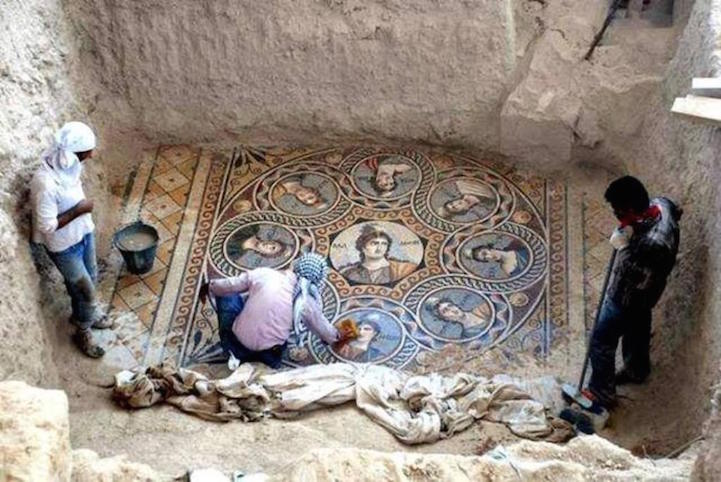In this color photograph, we observe an excavated underground room or cave set in what appears to be a desert or Middle Eastern locale. The gray, uneven walls form a rectangular space, viewed from above, with three individuals inside. Along the left wall stands a person in a white turban, matching white shirt, and jeans, gazing downward. The individual’s gender is indeterminate. On their knees, in the center of the room, another individual wearing a turban works intently, back facing us, cleaning a richly detailed rug. This exquisite carpet features a circular mosaic of faces and intricate patterns in shades of gold, gray, cream, and blue. Against the right wall, a third person stands upright, holding a long broom, also focusing on the cleaning task. Beside the kneeling individual, a pail filled with water and a sponge suggests meticulous care being taken to clean the rug. The image captures a moment of diligent craftsmanship and attention to detail within this secluded, dusty setting.